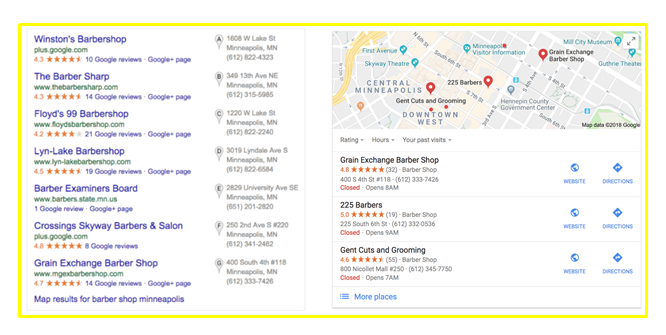The image is bordered by a yellow rectangle. On the left-hand side, a series of directories are displayed, each following a format that repeats seven times. Each entry begins with blue text indicating the name, followed by green text for additional details, and an orange star rating. On the third line of each entry, there is blue text specifying the number of Google reviews, sometimes mentioning a Google Plus page.

At the bottom of the directory listings, blue text reads "Map results for Barbershop Minneapolis." Next to each entry, in gray text, are the addresses and phone numbers, along with map icons labeled A through G. 

To the right, a visual map with three red map icons and three additional red dots is shown. Below this map, three barbershop locations are listed: "Green Exchange Barbershop," "225 Barbers," and "Gent Cuts and Grooming," each in black text. An orange star rating and gray text with the address and phone number are included beneath each location. The fourth line for each of these entries contains the word "closed" written in red text, indicating that all three locations are not currently open.